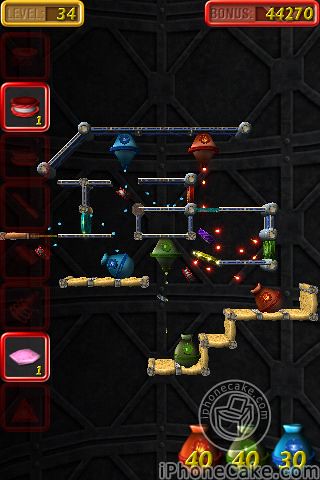This is a colorful screenshot of an addictive video game designed for iPhones, sourced from iPhoneCake.com as indicated in the lower right corner. The game features a two-dimensional, industrial-themed landscape with a black, square-patterned background interspersed with what appear to be cage-like designs. At the top left of the screen, a yellow box marks the player’s progress as level 34, while the top right corner displays a red box with a bonus score of 44,270 in yellow. The gameplay involves navigating through various levels showcased as staircases and avoiding hazards like lights being shot from cannons. In this particular image, there are three pipes, each holding jugs colored red, green, and blue, all marked with the number 40 in yellow. These pipes and jugs add to the challenge, with the objective to either collect or avoid them as part of the game’s mechanics.